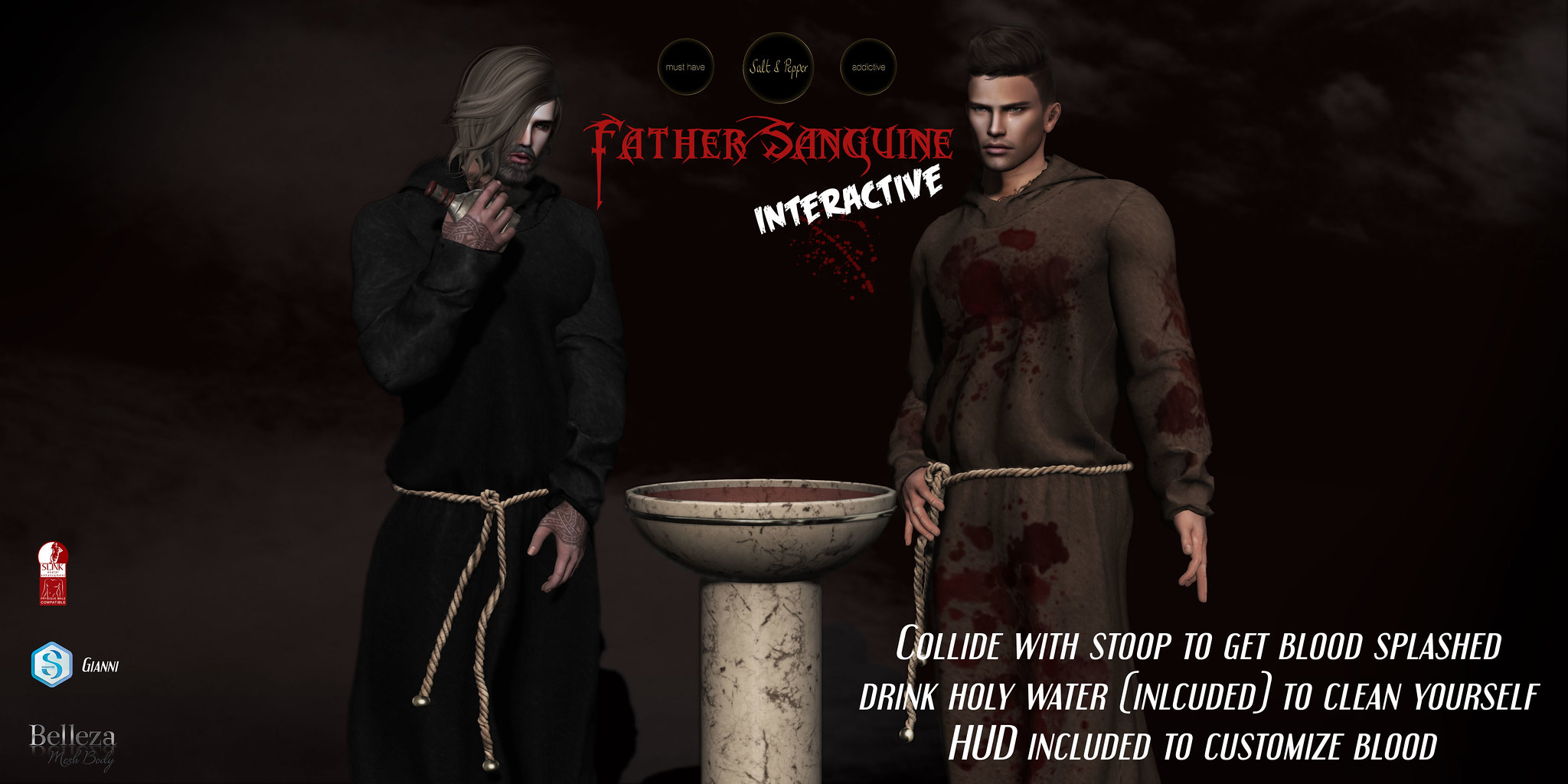The image appears to be a computer-generated graphic, reminiscent of a video game advertisement, presented in a landscape layout with a predominantly black background. At the center are two characters, both seemingly dressed in monk-like robes fastened with plain brown ropes. 

On the left stands an older white man with long, brown hair, a mustache, and a beard. He is clad in a black robe and has a tattooed hand holding up a bottle. To his right is a younger man, shorter and with darker skin and short dark hair. His attire is a brown robe with noticeable red splatters resembling blood stains, and he is clean-shaven.

Between the two characters stands a grey baptismal font, a bowl atop a pedestal, hinting at a ceremonial or ritualistic setting. Above this font, the red text reads "Father Sanguine," with "Interactive" in white below it. The bottom right corner features additional text that states, "Kaleido soup to get blood splashed, drink holy water included to clean yourself, HUD included to customize hood."

Three logos are situated in the bottom left corner: one marked with an 'S,' another reading 'BELLEZA,' and the third resembling a red globe or keyhole. The overall aesthetic and details suggest this is a promotional image for a video game, with elements emphasizing both mystical and interactive features.